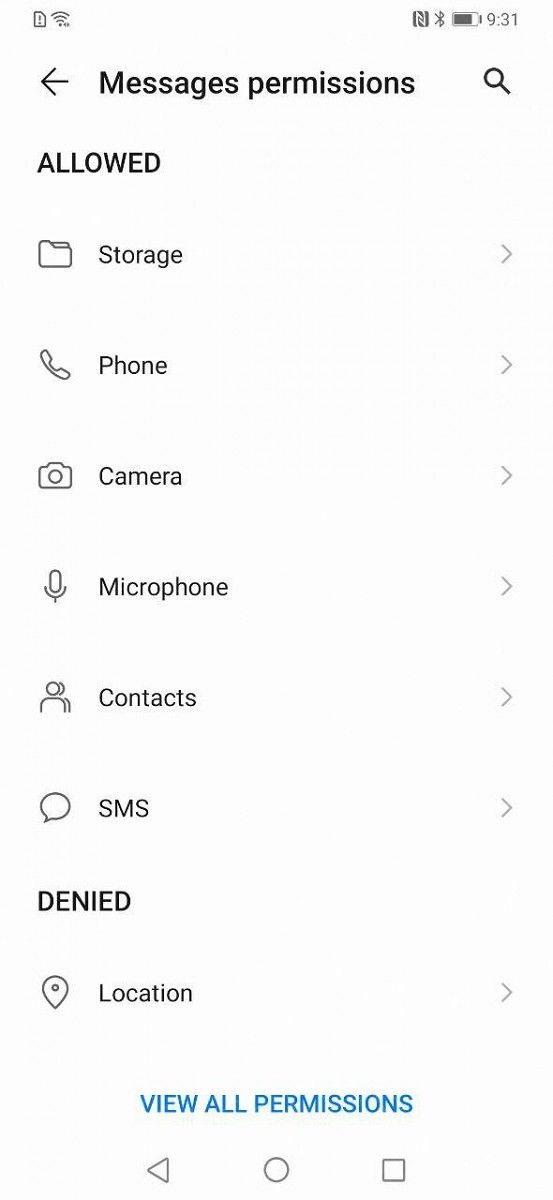This image features the screen of a cell phone displaying the permissions settings for a messaging app against a plain white background. In the upper left corner, there is a small box containing an exclamation point, symbolizing a notification or warning, followed by a wireless connection icon. The upper right corner showcases the Bluetooth icon, a battery icon, and a digital clock displaying 9:31. 

Directly beneath these status icons is a left-pointing arrow, adjacent to the bold text "Messages Permissions," accompanied by a magnifying glass icon, indicating a search feature. Beneath this header is the word "ALLOWED" in dark, capital letters, beginning a list of granted permissions, each with corresponding icons: 
- A folder icon labeled "Storage"
- A phone icon labeled "Phone"
- A camera icon labeled "Camera"
- A microphone icon labeled "Microphone"
- An image of two people labeled "Contacts"
- A speech bubble labeled "SMS"

Following these allowed permissions, the word "DENIED" appears in bold, uppercase text. Underneath this, a pin icon labeled "Location" is listed as denied.

Towards the bottom center of the screen, in blue uppercase letters, the text "VIEW ALL PERMISSIONS" prompts the user. Finally, at the very bottom, there are three navigation icons: a triangle pointing left, an empty circle, and an empty square. The screen is otherwise devoid of additional images, photographs, drawings, or varying background colors, maintaining a simple and uncluttered design.